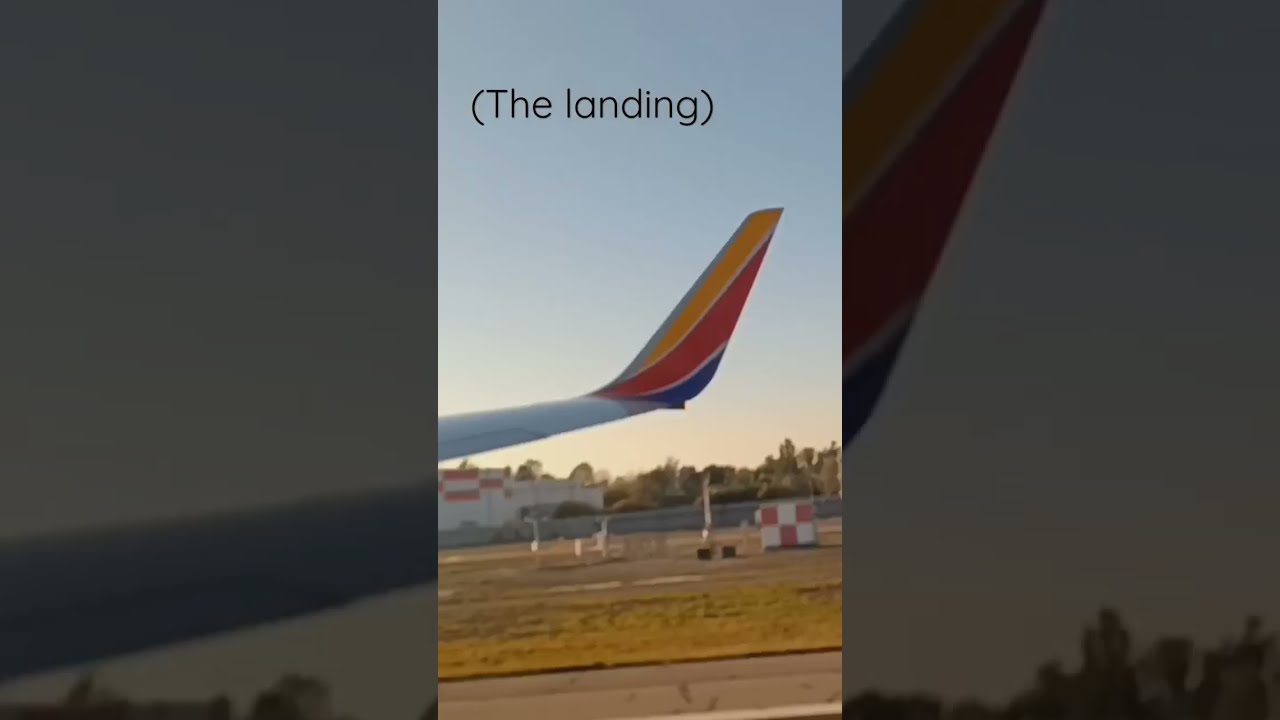This image captures the perspective from inside an airplane, looking out through the window at the tail end of the plane's wing, which is prominently featured. The wing tip, which resembles a sail or fin, displays the airline's logo with colors of orange (or yellow), red, and blue on its white body. At the top of the image, the phrase "the landing" appears in parentheses and black text. The plane appears to be either landing or taxiing on a runway strip bordered by a dry, grassy area, indicating that it might be fall. The sky is clear and predominantly blue, suggesting the time might be morning or evening, given the lack of bright sunlight. The background is quite small and slightly grainy, showing faint glimpses of buildings and possibly trees.